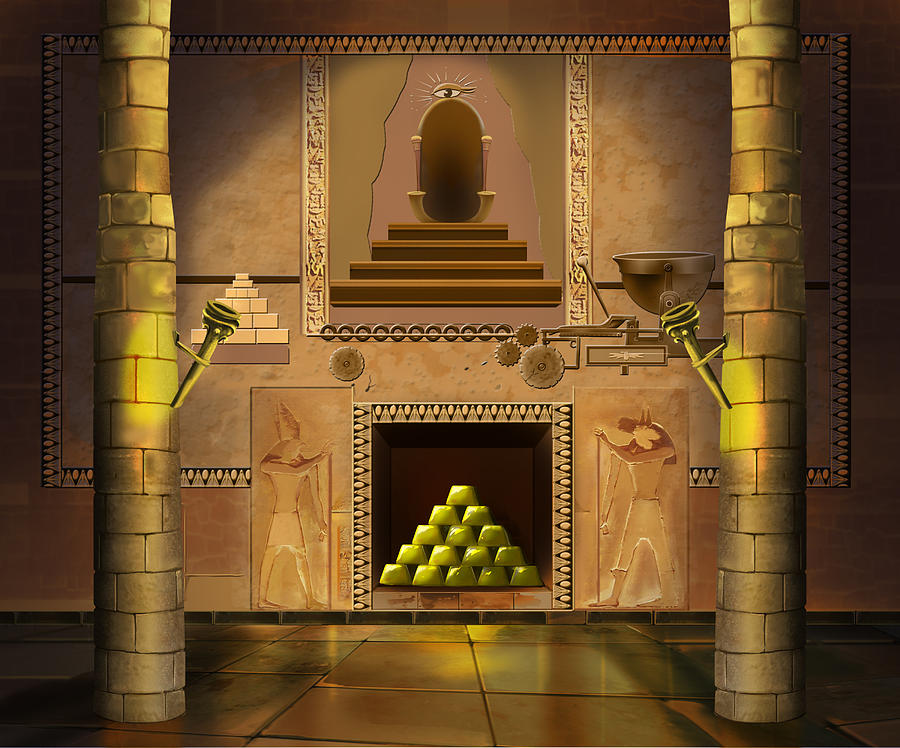This digital illustration depicts the interior of a pharaoh's tomb, masterfully rendered with predominant tones of gold, tan, and light stone gray. In the center of the image, a grand staircase, ascending to a mirror adorned with the Eye of Horus, captures immediate attention. This central element is framed by intricate carvings reminiscent of hieroglyphics and arrowhead patterns that embellish the top, left, and right edges, contributing to the image's ancient Egyptian aesthetic.

Flanking the staircase, there are statues of Egyptian gods adorned in traditional attire, each holding a staff. Below these sacred figures, the eye is drawn to an alcove filled with meticulously stacked gold bars, forming a pyramid shape. This treasure is nested within a vault-like opening, evoking the wealth and grandeur associated with pharaohs.

The setting is anchored by two robust, round columns made of stone that stand in the center of the room, one on each side. These pillars are equipped with brackets, originally designed for holding torches. Above the golden bars, partially visible gears and a lever suggest the presence of a possibly intricate locking mechanism, balancing the artistic and functional aspects of ancient tomb architecture.

The color palette transitions smoothly from gold to red-tinted tan, creating a coherent yet vibrant atmosphere. The floor, seemingly tiled with gold, reflects the ethereal glow, enhancing the overall opulence of this hidden chamber. As a whole, the illustration eloquently captures the mystique and splendor of an ancient Egyptian pharaoh's secret domain.